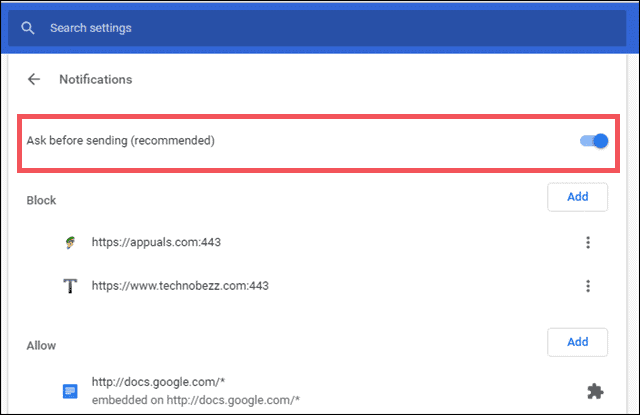**Caption:**

The image portrays a comprehensive notification settings page. At the top, a blue rectangular banner features a darker blue search box with a white magnifying glass icon, labeled "Search settings." Below this, a section on a white background with a light gray border displays a bold, dark gray arrow pointing left next to the word "Notifications."

Further down, black text reads "Ask before sending" with "(recommended)" in parentheses, accompanied by a blue toggle switch outlined in a thick red rectangle, indicating it is on. Below this, "Block" is listed in black text alongside a white button with blue text and a light gray border reading "Add."

Subsequently, two items are listed with menu options on the right denoted by three vertical dots. The first item includes an unidentifiable icon and the URL “https://appuals.com:443,” followed in the next row by a T-shaped logo and the URL "https://www.technobez.com:443." Each item has a corresponding "Allow" button with a white background, blue text, and a light gray border on the right.

The final section lists "http://docs.google.com/&" twice, with an accompanying blue document icon on the left and a dark gray puzzle piece icon on the right.